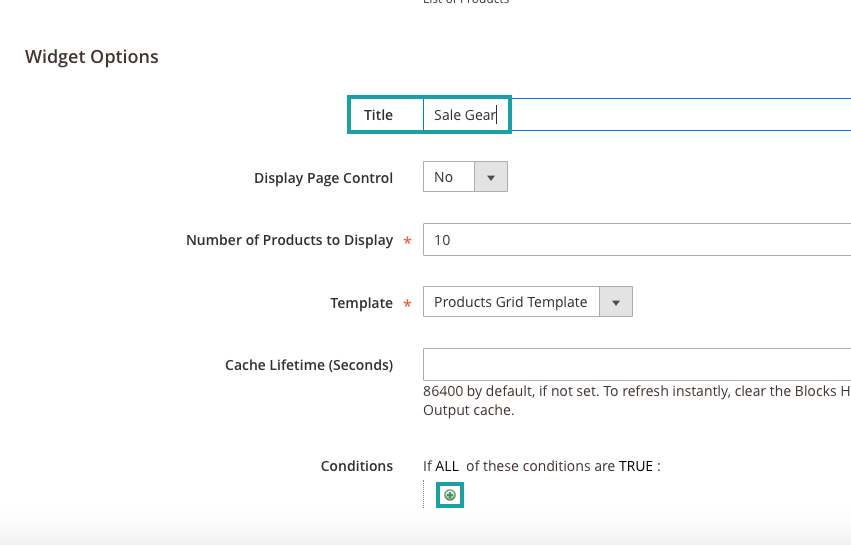The screenshot depicts an interface, likely from a desktop or mobile device, against a white background. In the top-left corner, the title "Widget Options" is visible in black text. 

On the right side, a section is highlighted with a teal box labeled "Sales Gear." Directly beneath this section, the term "Display Page Control" appears, accompanied by a dropdown menu currently set to "No."

Further down, the option "Number of Products to Display" is present, marked with a red asterisk. The value "10" has been input. Below this, another option labeled "Template" also features a red asterisk, with its dropdown menu showing the selection "Products Grid Template."

The next option is "Cache Lifetime (seconds)," with an input bar containing the value "86,400" and a note indicating this as the default unless set to refresh instantly. Additionally, it mentions "Clear the Blocks' Output Cache."

At the very bottom, the section titled "Conditions" appears. Beside this title, a statement reads, "IF ALL OF THESE CONDITIONS ARE TRUE," with "ALL" and "TRUE" in uppercase. Directly below this statement, a turquoise-colored box with a circle in the center is displayed.